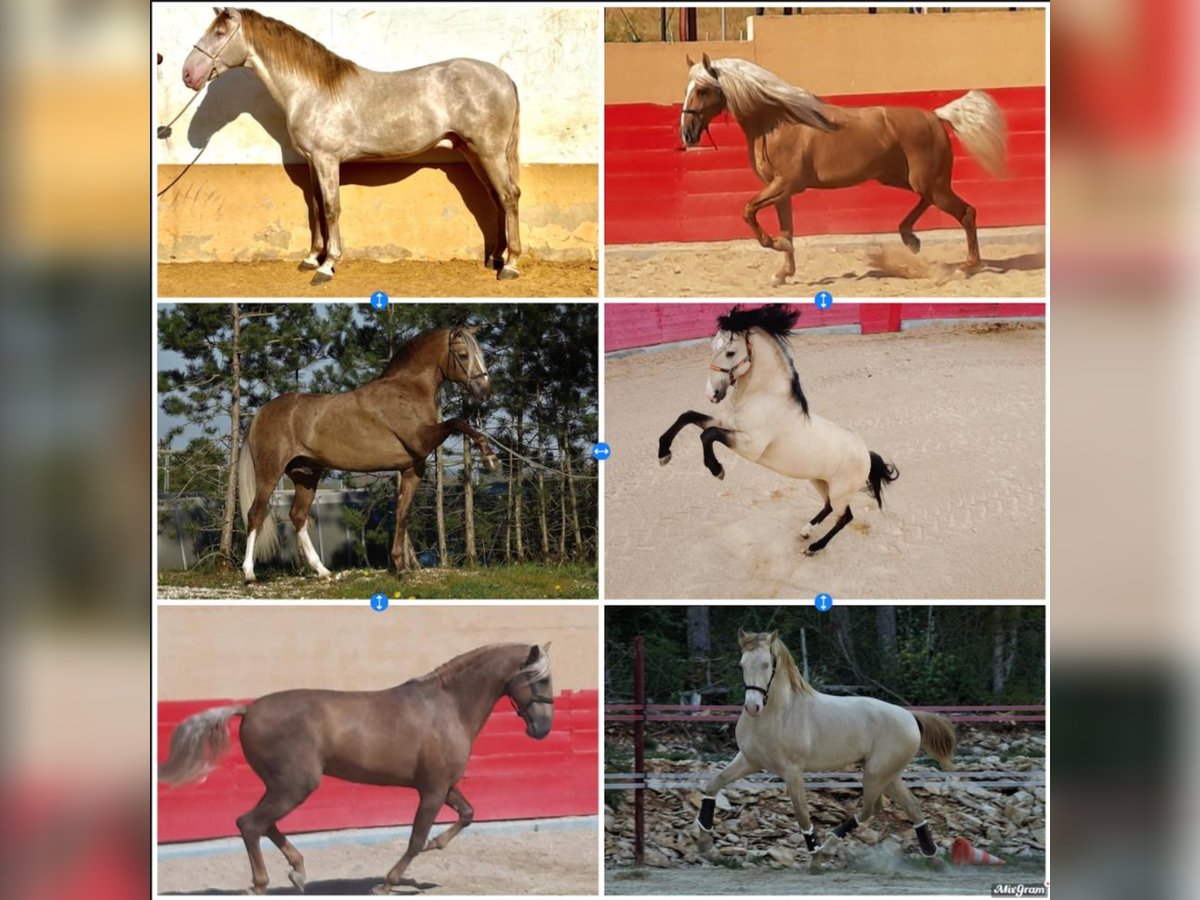The image is a collage featuring six distinct photos of horses, arranged in two columns and three rows within a square frame that has thick, blurry borders on the left and right sides. The borders blend colors like red, white, black, yellow, and gray, creating a textured effect.

Starting from the top left, the first image shows a gray horse with a brown mane, standing still and facing left. It has a rope coming from the left side, and it is set against a background with a white upper part and an orangish-tan lower part. 

To its right, the top right image depicts a brown horse with a white mane and tail, trotting across sandy or dirt ground. Its left front hoof and back right hoof are raised as it moves from right to left, with a backdrop featuring a red and cream-colored wall.

In the middle row, the left image captures a brown horse with white markings, including white socks and a blondish tail. This horse stands on grass with trees visible in the background. The middle right image features a white horse with a black mane and legs, mid-air with its front hooves raised. The horse appears to be in a rodeo ring, with a red wall and a small pink fence in the distant background.

On the bottom left, a brown horse with a brown mane and tail is shown trotting left to right, again against a red and cream-colored wall, likely on dirt ground. The final image on the bottom right displays a white horse with a brown mane and tail, running from right to left through an outdoor course. There is a fence and trees visible in the background, highlighting the natural setting. 

Overall, the horses are depicted in various poses and environments, including standing still, trotting, and rearing up, each adding unique characteristics to the vibrant collage.